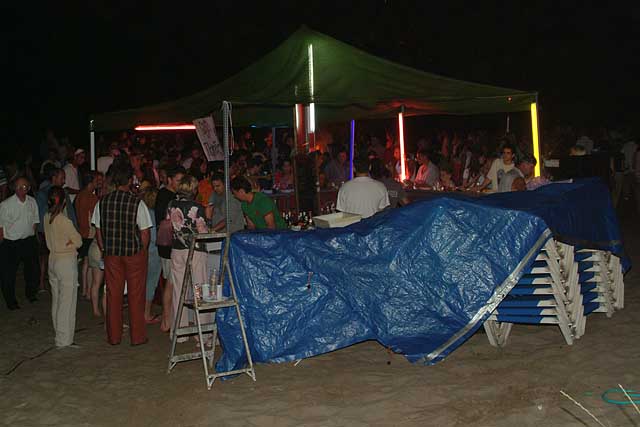The image captures an outdoor evening event, likely a lively night-time party or street fair, set under a dark sky. The central focus is a large tent, supported by metal poles and adorned with vibrant neon lights, creating a festive atmosphere. Crowds of people, estimated in the hundreds, surround the tent, suggesting a popular gathering. The terrain appears sandy, indicating a possible beachside location, although everyone is fully dressed, ruling out a beach scene.

Underneath the tent, bottles and other bar-like accoutrements imply that it serves as a bar, enhancing the celebratory vibe. In the foreground, a blue tarp covers a set of beach recliners, and nearby stands a metal stepladder with drinks placed on its steps. The attendees, visible in the dim light, include men and women enjoying the event; notable figures include a man in red trousers, a plaid vest, and a white shirt, standing near a woman in tan pants and a pink shirt. The scene exudes a sense of nocturnal revelry and communal enjoyment amidst the softly lit, neon-glowing setup.